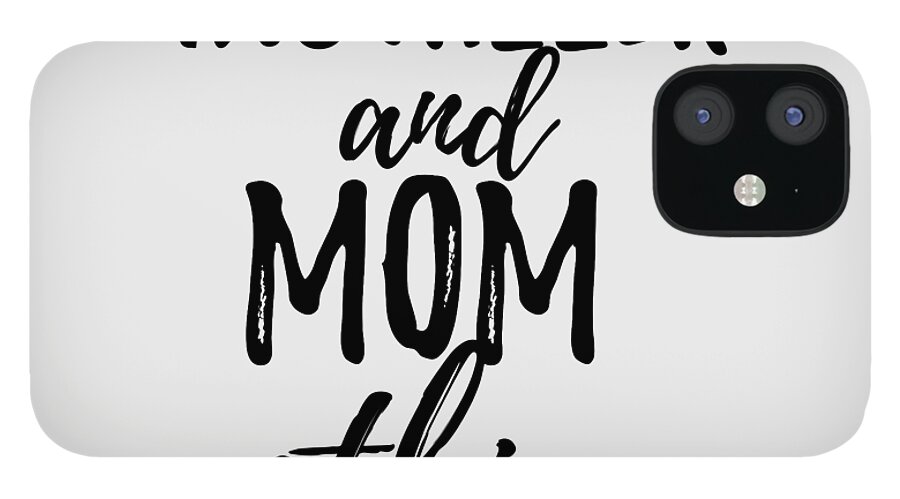The image depicts an advertisement for a matte white smartphone case, specifically designed for a newer iPhone model characterized by its round edges and triple-camera setup. The camera array—comprising a telescopic lens, a wide-angle lens, and an additional sensor subtly blending into the black rectangular camera cut-out—also features a light-colored LED flash nestled among them. The phone is shown on its side against a clean, white background, enhancing the advertorial style. Dominating the middle of the case is textured black cursive text that reads "AND MOM" in all caps, with additional, partially visible cursive letters peeking out from both above and below this central phrase. The text has an inked texture with some white flecks indicating incomplete coverage.